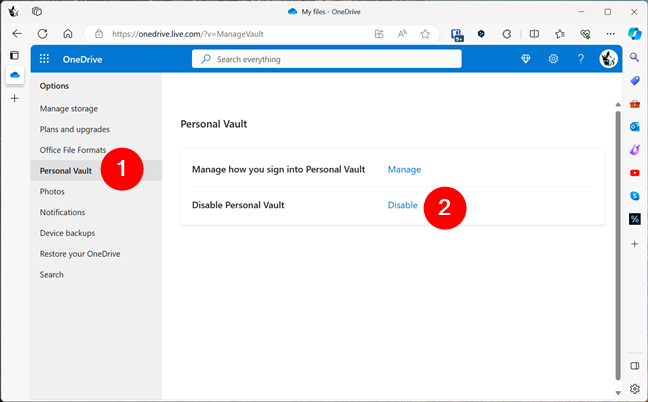This is a detailed screenshot of a computer application interface, specifically the OneDrive dashboard. The interface features a light gray header and sidebars on either side. 

In the center of the top header, there is a distinctive multi-colored blue cloud icon. Directly to the right of this icon is the text "My Files - OneDrive," prominently displayed in black with capitalized letters "O" and "D."

On the top left, there are two dark gray icons. Below these and on the sidebar, there are several more icons arranged vertically: a gray left-pointing arrow, a gray calendar icon, a white box icon with rounded corners casting a light gray shadow. This white box icon also features a multi-colored blue cloud in its center. Beneath this, there is a dark gray plus icon.

Adjacent to the left-pointing arrow, on the top header, there is a dark gray refresh icon. To the right of the refresh icon, a dark gray house icon is visible. Next to this house icon is a URL bar shaped like an elongated white pill. On the far left of this bar, there is a light gray lock icon, followed by the text "HTTPS://" in light gray. Continuing in black text, the URL reads "OneDrive.live.com," followed by "V=manage vault" in light gray text with capital "M" and "V."

At the far right of the search bar, there is an icon resembling three dark gray boxes forming an "L" shape with a dark gray plus sign in the top right corner. To the right of this icon, there is a medium gray "A" with a percentage symbol next to it, and finally, to the right of this, a medium gray star icon.

This detailed visual description provides a comprehensive understanding of the OneDrive application's user interface elements visible in the screenshot.